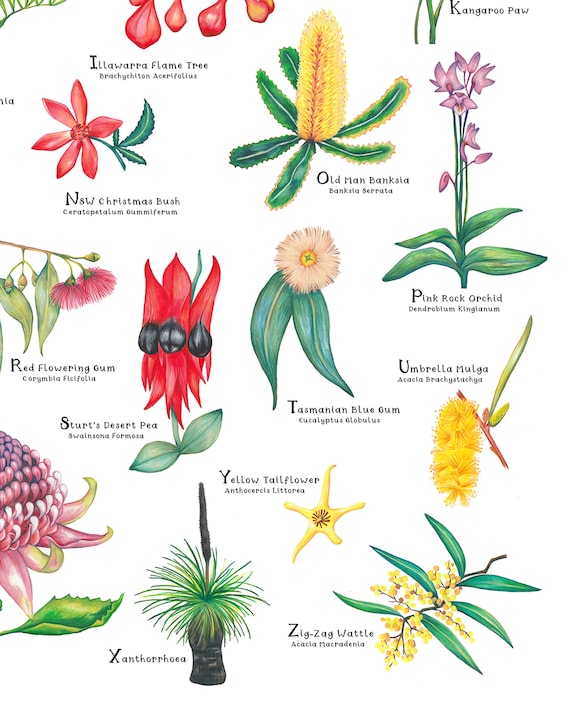This image is a detailed, colored drawing of various flowers and plants, meticulously labeled with both common and scientific names on an off-white or ivory background that resembles wallpaper or illustrations from historical botanical texts. In the center, there's a Tasmanian Blue Gum, a pink flower with a red interior and green leaves. The lower right features a Zigzag Wattle, displaying clusters of yellow flowers extending from a stem with leaves on either side. Towards the center bottom, sprouting from a vase, is a Xanthoara, showcasing green sprouts and a taller central stem. The upper right depicts an Umbrella Mulga, a tubular yellow flower hanging from a red stem, and nearby in the same area is a Pink Rock Orchid, characterized by its green stem, leaves at the base, and pink and purple blooms at the top. To the center left is Sturt's Desert Pea, a striking red flower with three dark purple or almost black bulbs on its front, emerging from green leaves. In the upper left corner, the NSW Christmas Bush is shown with a red flower growing out of a simple green leaf. Other plants include Old Man Banksia, Kangaroo Paw, Illawarra Flame Tree, and several others, each vividly rendered in colors like red, yellow, pink, and green, giving a comprehensive and aesthetically pleasing botanical overview.